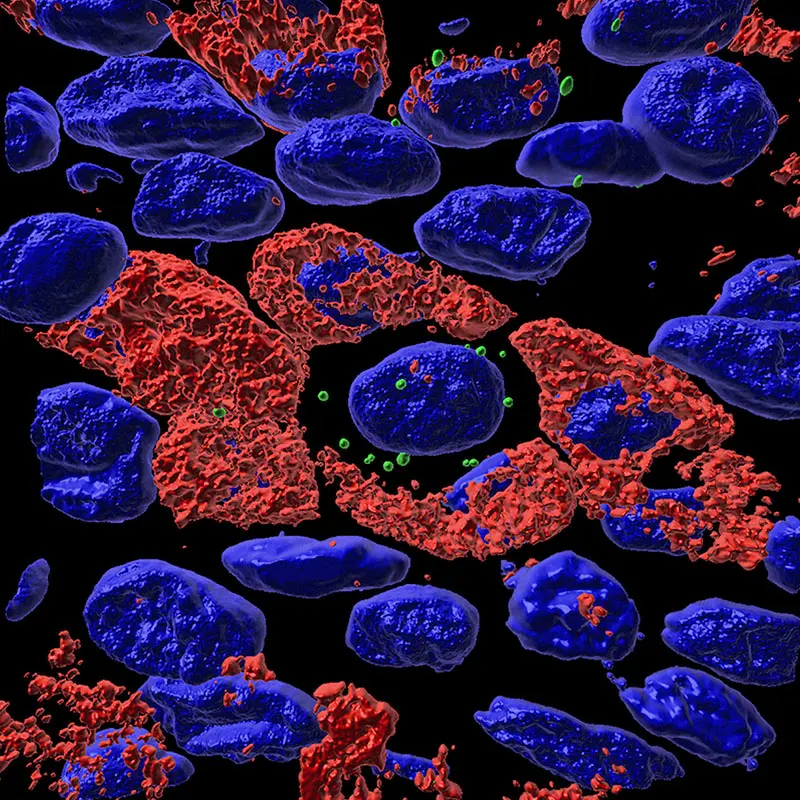In this computer-generated or machine-scanned medical image, various cell-like shapes appear against a black background, illuminated in bright neon colors. Predominantly, there are numerous oval and circular blue blobs, which are reminiscent of cells or particles. Interspersed among these blue shapes are vivid orange, coral-textured blobs with a liquidy appearance that weave through and surround the blue structures. The center of the image features a singular, isolated blue blob encircled by tiny green spheres, which are sparsely scattered throughout the composition, with a higher concentration around the solitary blue shape. The entire scene is bathed in an ultraviolet light that accentuates the vivid hues, creating a complex pattern that resembles a cosmic or microscopic landscape, filled with floating, rock-like molecules.